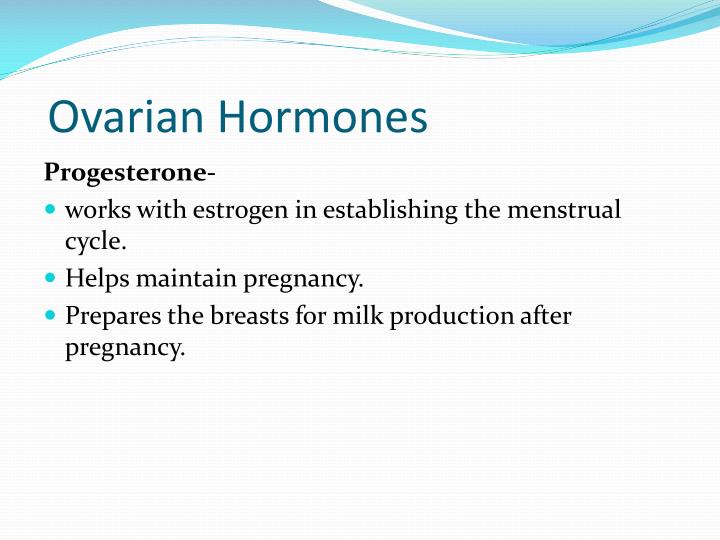The image appears to be an educational slide or digital graphic, likely created using PowerPoint. The background is a clean white-grayish color, and across the top, there is a decorative wavy pattern that transitions from light blue to darker grayer blue, about an inch wide. Below this wave, in all caps and large dark blue text, the title "Ovarian Hormones" is prominently displayed. Underneath, in bolded black text, "Progesterone" is written. The main content is presented in three bullet points, each in a light blue font. These bullet points detail the functions of progesterone: it works with estrogen to establish the menstrual cycle, helps maintain pregnancy, and prepares the breasts for milk production after pregnancy. The text is centrally positioned and easily readable, contributing to the overall clarity and educational focus of the slide.